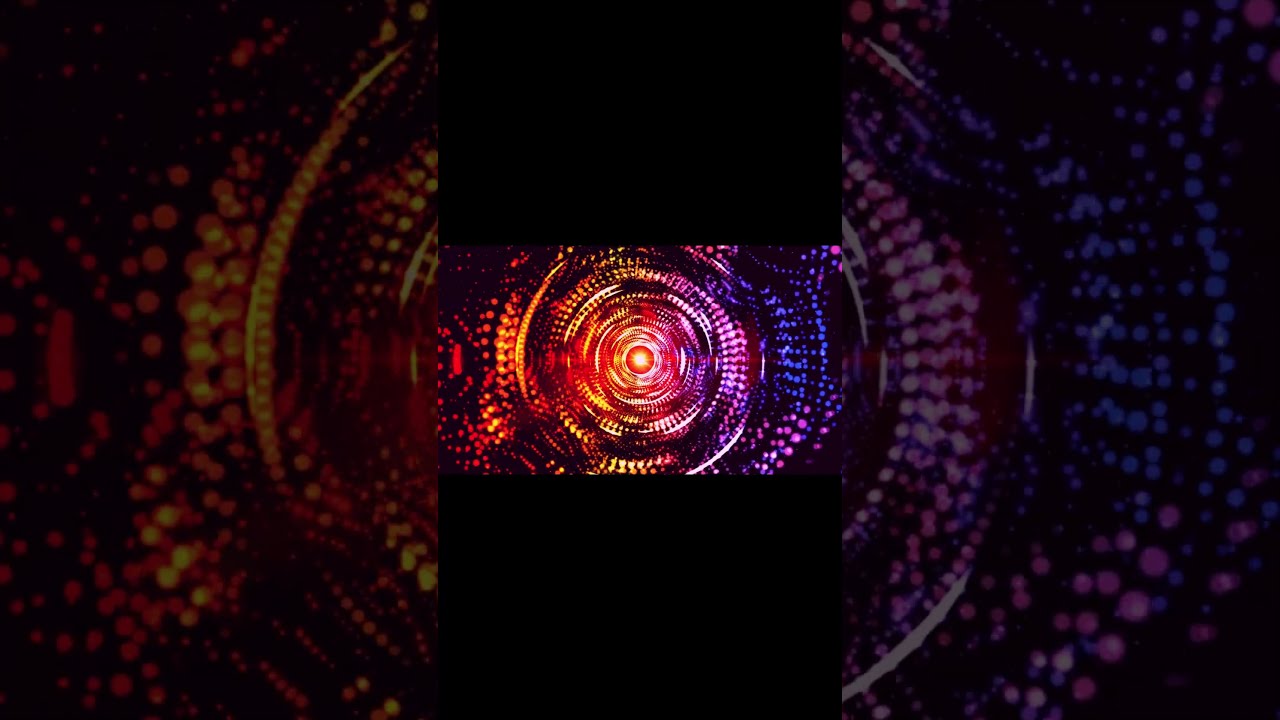The image features a vibrant circular design, resembling the eye of HAL 2000 from "Space Odyssey 2001," with a striking ripple effect. The outer edges of the design are faded black, transitioning into vivid colors toward the center. The central portion is a radiant yellow, encircled by an orange ring, composed of variously sized dots. Surrounding this core are concentric circles in a spectrum of colors: gold and dark red hues dominate the left side, while pink and dark blue shades fill the right. This intricate design is framed by large black borders at the top and bottom, occupying more than a third of the image each, creating a contrasted backdrop that magnifies the central vibrant pattern. The side sections of the image are darkened and magnified, enhancing the focal point's kaleidoscopic appearance with rings of purple, pink, orange, yellow, blue, and lavender hues radiating outward.